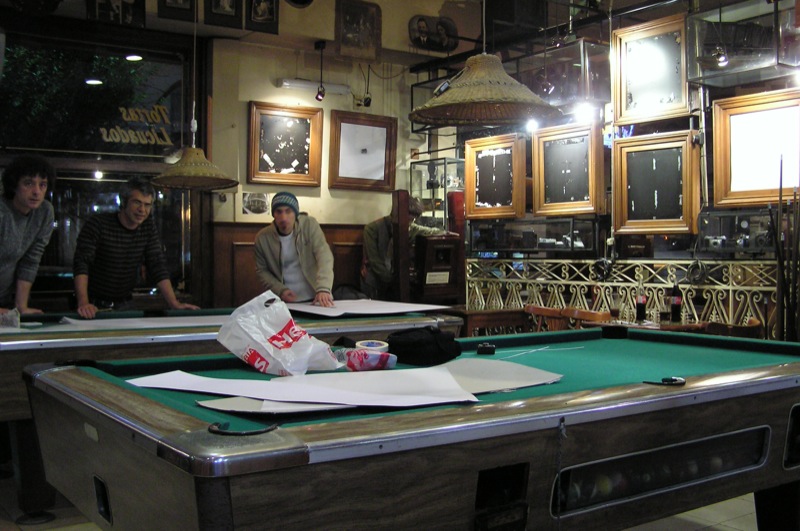The photograph is a detailed, colorful depiction of an interior pool hall, taken from a landscape orientation. The foreground prominently features a green-felted billiard table with its longest side facing the viewer and a corner pocket positioned in the bottom left. The walls to the back and partially to the left are adorned with numerous empty, ornate wooden frames, traditionally used for oil paintings, now showing black backgrounds and remnants of stickers where artwork once hung.  

In the background stands another pool table where three men are leaning weightily onto it, their attention absorbed by large white sheets of paper spread before them. The men, possibly the owners, sport distinct attire: one in a gray shirt, another in a striped gray and black sweater, and the third in a white shirt beneath a cream overcoat, topped with a knit green cap. Additionally, there's a faintly visible fourth individual, slightly obscured by a wooden beam, who could either be standing or sitting. 

The scene is softly lit by wicker lamps hanging from the ceiling, illuminating the room filled with scattered plastic bags and assorted papers, possibly suggesting the establishment is under setup or renovation. The captured moment exudes a quiet anticipation, with the men engrossed in their plans while surrounded by the quirky decor of mismatched, empty frames.